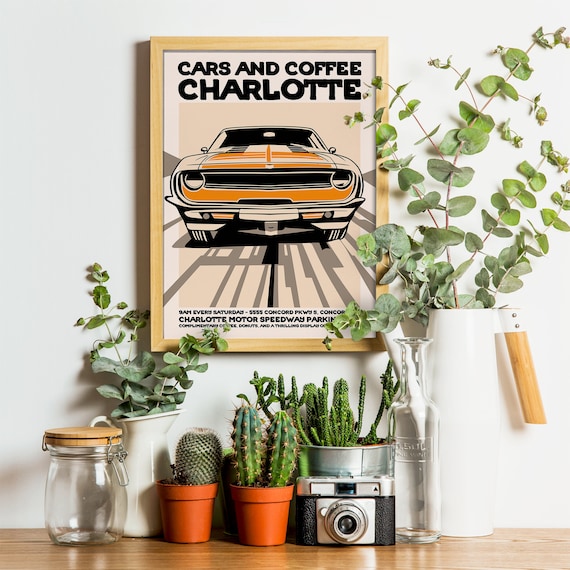This photograph captures a visually intriguing setup featuring a rustic wooden countertop adorned with various plants, set against an all-white wall. Central to the image is a framed poster promoting "Cars and Coffee, Charlotte," an event at the Charlotte Motor Speedway. The focal piece features the front end of a muscle car, artistically depicted in shades of white, light orange, and darker orange, enclosed in a light blonde wood frame. 

Below the poster, the countertop is populated with an assortment of potted plants and cacti. From left to right, there is a clear mason jar with metal clips, seemingly empty. Next to it is a white flower pot with green stems, followed by a small plastic pot housing a single cactus. Further along, there’s another pot with two elongated cacti, positioned beside a vintage camera resting on the countertop. Behind the camera, a silver aluminum bucket contains a cluster of stringy cacti, completing the plant arrangement.

On the far right, a larger white cylindrical vase filled with lush greenery offers additional contrast to the scene. The entire arrangement presents an interesting juxtaposition between the vibrant promotional poster and the natural elements of the plants and cacti, creating a unique and visually captivating composition.